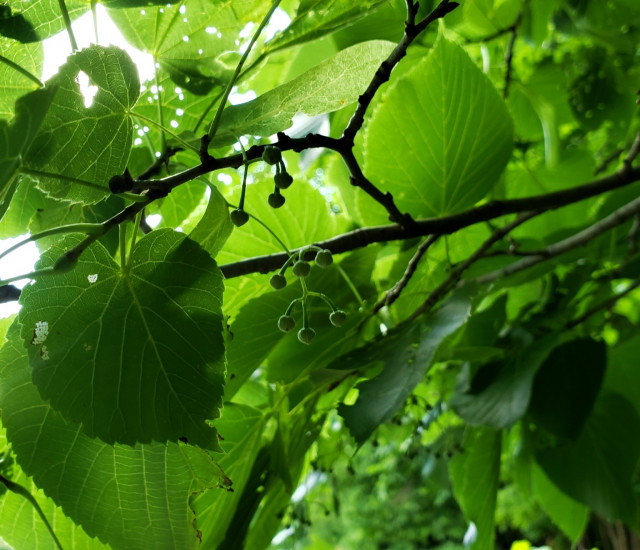This detailed photograph captures an up-close view of a tree adorned with heart-shaped, serrated leaves showcasing intricate details. The leaves exhibit lighter green veins contrasted against their darker green background, and some display holes resulting from insect damage. Through these holes, bright sunlight, appearing white, filters down from the sky, casting a varied illumination across the scene. The camera angle is from the underside of the tree, creating a backdrop of the bright sky through the canopy.

Highlighted in the image are small, twig-like branches extending from the right side to the left. Hanging from these branches are clusters of small, unripe fruits, each grouping containing three to four green, round yet asymmetrically shaped berries. The fruits are positioned centrally within the photo, with their green hues blending into the leafy surroundings.

Absent of animals, people, or text, the focus remains solely on the natural beauty and intricate details of the tree’s foliage and developing fruits. The sun's position at the top left creates a play of light and shadow, adding depth to the photograph while casting darker tones in the bottom right areas where the leaves and branches grow denser.